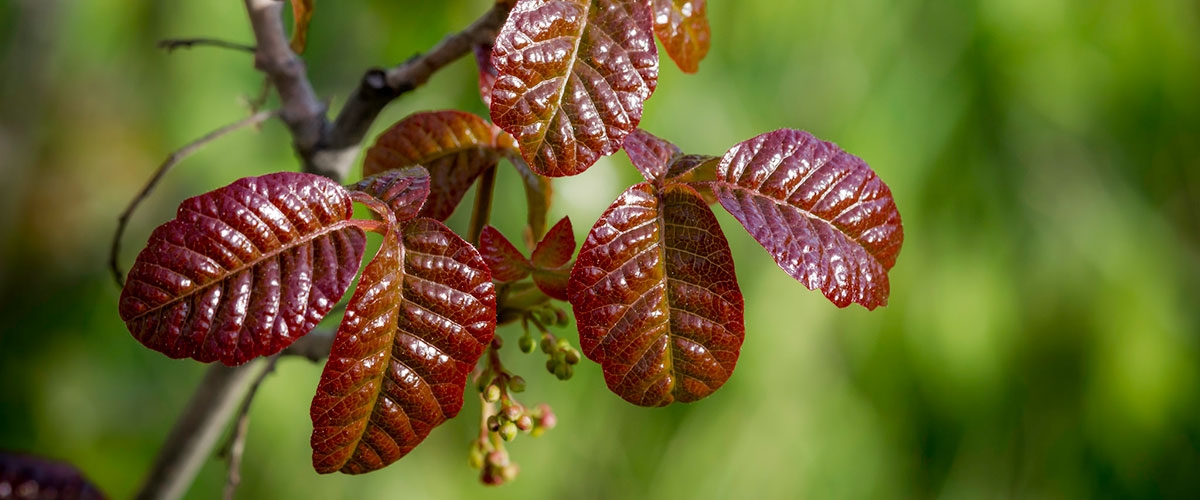An outdoor, full-color photograph captures a close-up of a tree branch with distinct deep red, oval-shaped leaves, utilizing natural daylight. This horizontally rectangular image features a blurred background filled with various shades of green vegetation, providing a soft contrast to the sharply focused branch. The branch originates from the bottom left corner, extending diagonally and branching into two directions, one upward to the left and the other to the right, both exiting the frame. Prominently, six red leaves, with visible ridges and veins, are positioned around this branch. One leaf extends back and to the left, one hangs down to the right partially folded, and another lies above these going slightly upward to the right. Additional leaves are positioned upward and to the left of these, with one leaf entering from the image's top edge. The lower section of the branch displays several unopened buds, suggesting early spring. Light glints off the surface of the open leaves, enhancing their rich color and texture. An oval-shaped, darker object is partially visible in the lower left corner, adding to the composition's intrigue.